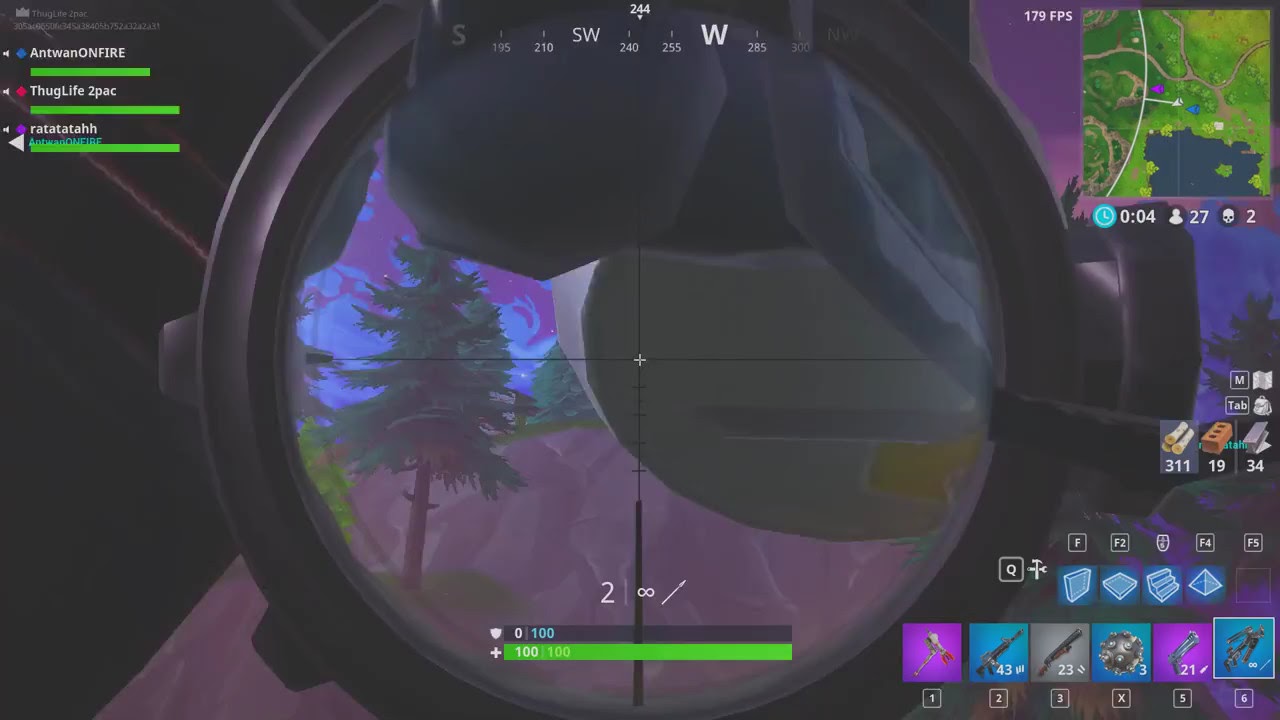The image is a detailed screenshot from a video game, likely Fortnite, showcasing the perspective through a sniper rifle scope. The crosshairs are centered on what appears to be rocky terrain with some pine trees, a gray stone hill, and a sky filled with purple and blue swirling clouds. Taking up the top portion of the screen is a compass pointing between southwest and west. The top right corner contains a mini-map with road and greenery details. The HUD is rich with game information: a frame rate of 179 FPS, a clock reading 0:04, and a player count of 27. At the bottom left, player health and shield stats show one player at 0/100 for shield and 100/100 for health, while another player has 100/100 for both. The right side displays a weapon selection interface with various weapons highlighted in different colored backgrounds. Visible usernames—Antoine, On Fire, Thug Life 2-Pack, and Ratatouille—are presumably teammates, with corresponding health bars indicating their statuses. The scope’s crosshairs obscure a white, rounded object, though details are indistinguishable.